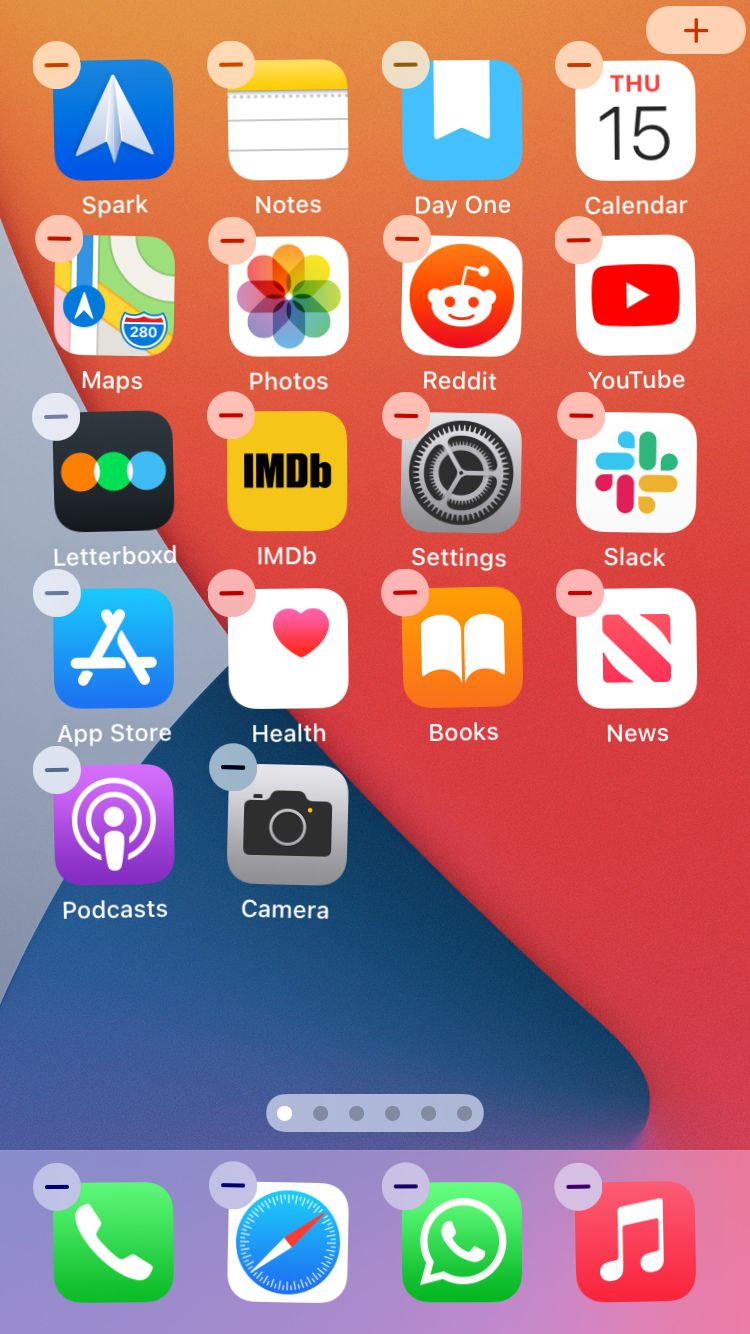The image features an iPhone screen displaying various app icons. The icons are currently in the "jiggle mode," indicating that they can be moved or deleted; each icon has a small negative sign in a circle at its top left corner. This mode is typically activated when the user holds down on an app icon, causing all icons to start shaking and allowing for reorganization or deletion. 

The background of the screen is a vibrant gradient with hues of orange and red at the top, transitioning to blue in the lower left, and gray in the upper left. The app icons are somewhat tilted and appear misaligned due to the jiggle mode. 

The list of apps includes: Spark, Notes, Day One, Calendar, Maps, Photos, Reddit, YouTube, Letterboxd, IMDb, Settings, Stack, App Store, Health, Books, News, Podcasts, and Camera. At the bottom dock, the phone displays four primary apps: Phone, Safari, Messages, and Apple Music. 

To exit this mode and stop the icons from shaking, one can press the Home button, which will also remove the negative signs and return the screen to its standard layout.